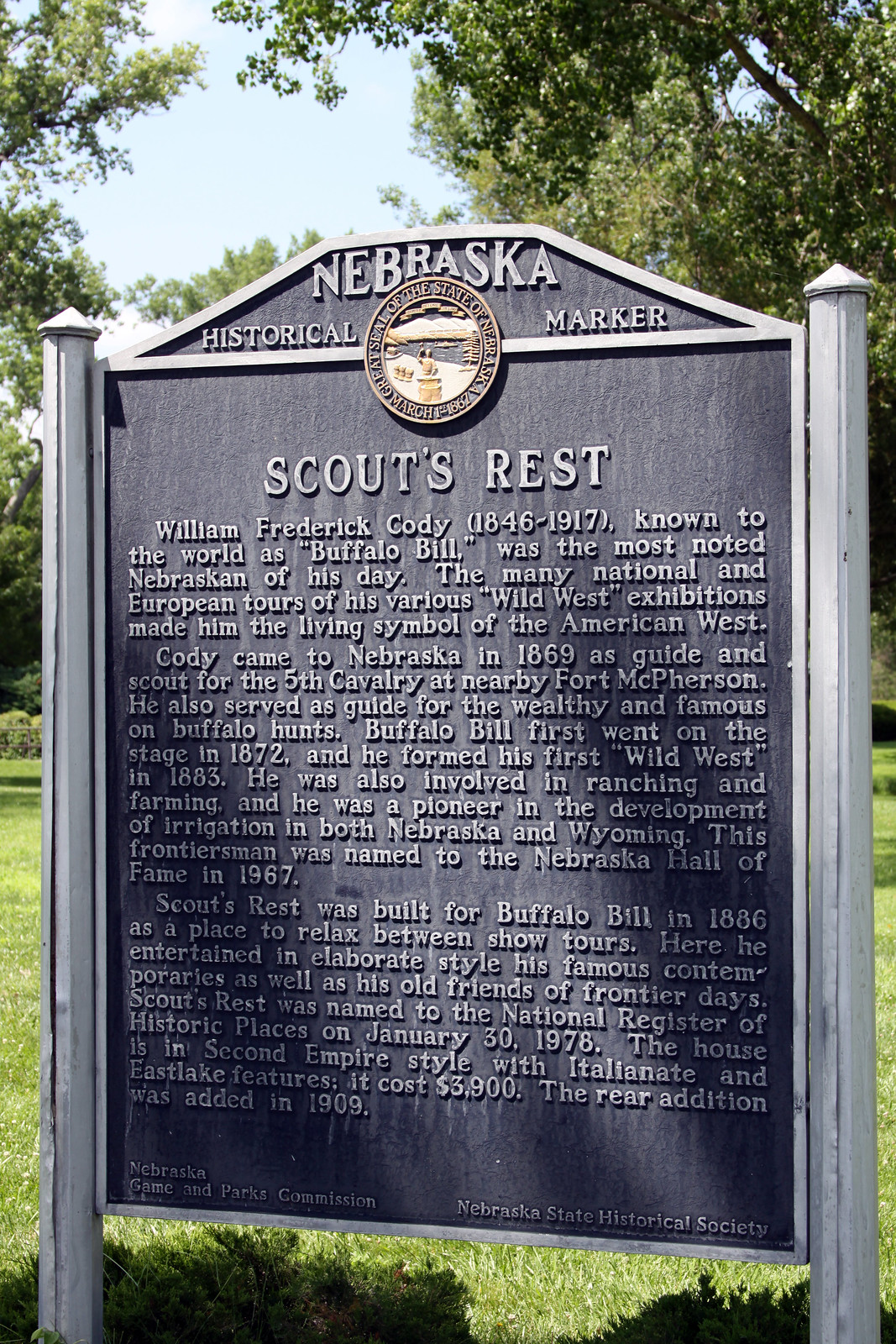The image depicts a historical metal sign set against an outdoor backdrop of trees, grass, and bushes, suggesting it is located in a park. The sign has a dark gray background with raised text. At the top, it reads "Nebraska Historical Marker," with a circular disk positioned between the words "Historical" and "Marker." This disk features a ring of text encircling a landscape image, possibly representing the state crest of Nebraska.

Below the crest, the title text reads "Scouts Rest." The following paragraphs provide detailed historical information about William Frederick Cody, widely known as Buffalo Bill, who was a prominent figure from Nebraska. Born in 1846 and passing away in 1917, Buffalo Bill gained fame through his various Wild West exhibitions, which toured nationally and internationally. 

The sign details his arrival in Nebraska in 1869, where he served as a guide and scout for the 5th Cavalry at Fort McPherson, and later became a guide for affluent and notable individuals on buffalo hunts. Buffalo Bill made his stage debut in 1872 and established his first Wild West show in 1883. He was also a rancher, farmer, and pioneer in irrigation development in Nebraska and Wyoming. In recognition of his contributions, he was inducted into the Nebraska Hall of Fame in 1967.

"Scouts Rest," Buffalo Bill's home built in 1886 as a retreat between show tours, is described as a venue where he hosted both famous contemporaries and old frontier friends in elegant fashion. The house, exemplifying Second Empire style with Italianate and Eastlake features, cost $3,900 to build and had a rear addition added in 1909. It was listed on the National Register of Historic Places on January 30, 1978.

The sign is supported by two metal columns on either side, each topped with small conical shapes.